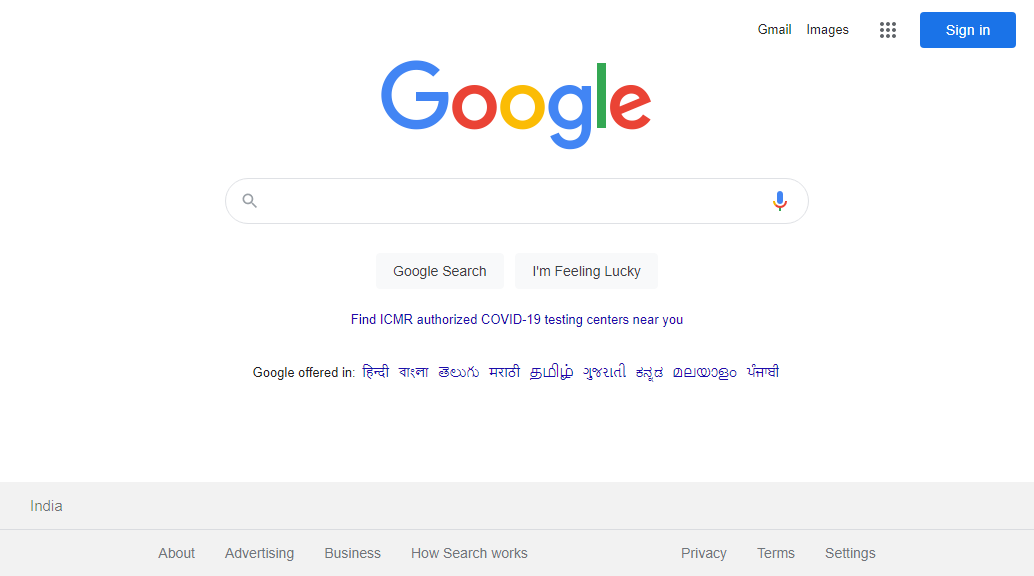This image is a screenshot of the Google Search homepage. In the top right corner, there are links and buttons including 'Gmail', 'Images', and a grid icon providing access to all Google Apps. Further along the top right, there's a prominent blue 'Sign In' button. 

Centrally positioned on the page is the iconic Google logo, directly above an expansive search box which features a microphone icon for voice search functionality. Below the search box are two distinct buttons labeled 'Google Search' and 'I'm Feeling Lucky', which offer different search experiences based on user preference.

Beneath these buttons, there is a link to find ICMR-authorized COVID-19 testing centers, a feature highlighting Google's commitment to providing relevant and timely information to its users. 

The page also caters to the linguistic diversity of India, as indicated by the text offering Google in various Indian languages. The location of the searcher is confirmed by the mention of 'India' in the bottom left corner of the screen.

The footer section of the homepage includes additional links for 'About', 'Advertising', 'Business', 'How Search Works', 'Privacy', 'Terms', and 'Settings', providing quick access to important information and settings.